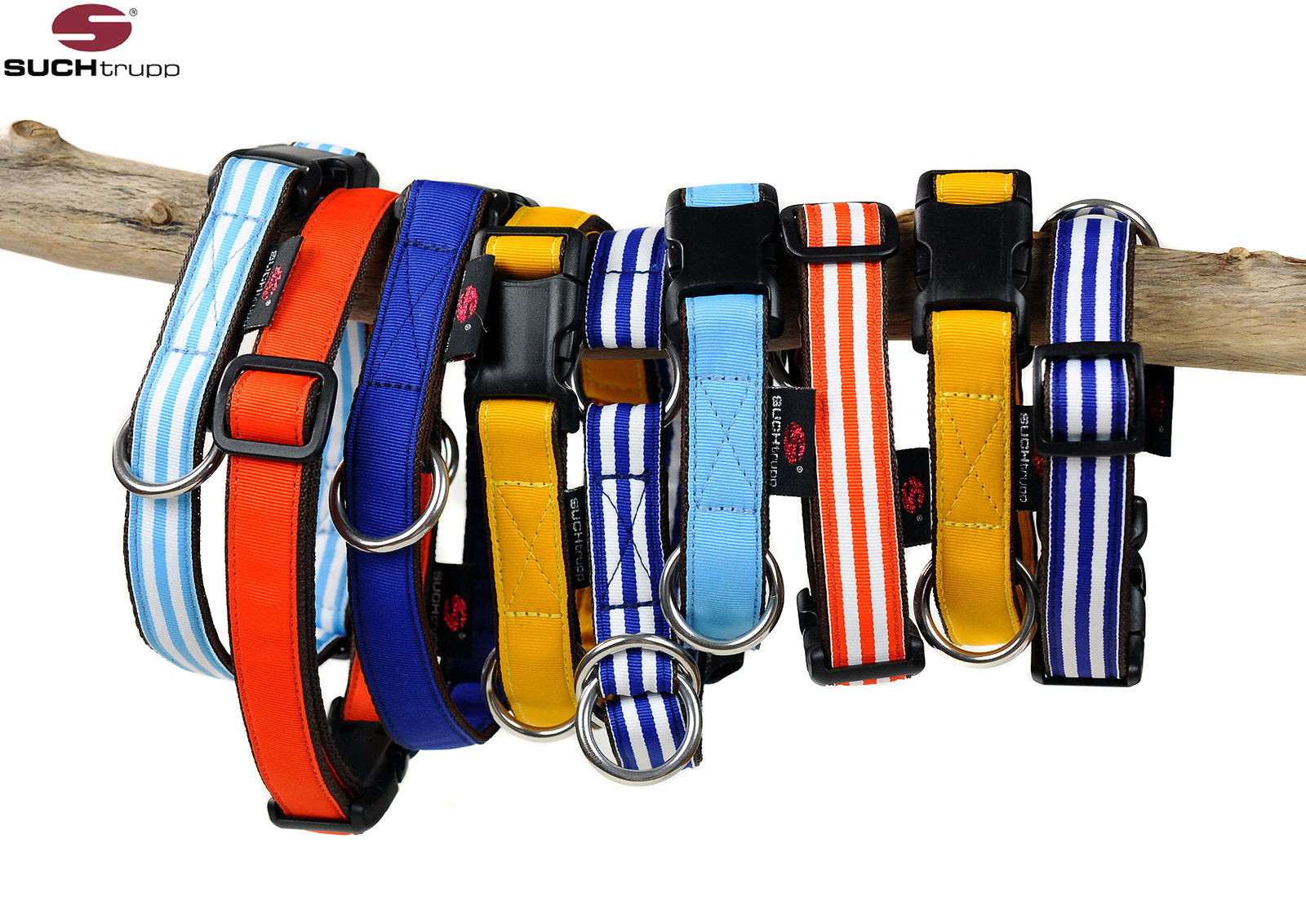This stock image portrays nine colorful dog collars hanging from a light wooden tree branch that stretches horizontally across the center of the frame. Each collar loops around the branch, displaying various vibrant color patterns including striped combinations of blue and white, orange and white, as well as solid bands in dark blue, orange, yellow, light blue, and more. The collars are equipped with black buckles and feature silver steel loops designed for attaching leashes or tags. The background is a pure, well-lit white, emphasizing the colors and details of the collars. In the top-left corner, a distinctive logo appears: an eccentric-shaped 'S' encircled within a maroon oval, accompanied by the brand name "Suchtrupp" in black text.